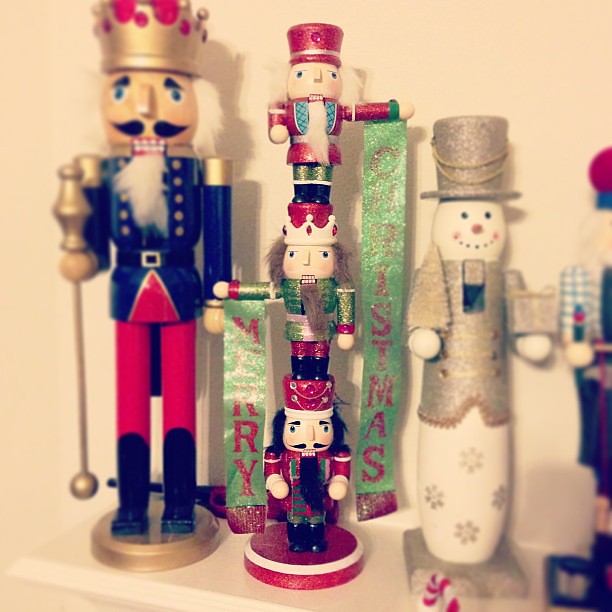In this festive image, a collection of Christmas decorations is artfully arranged. On the left side, there is a tall, regal nutcracker adorned with a royal blue jacket, red pants, black boots, and a golden-yellow base. It sports a red and gold crown, a black mustache, blue eyes, red lips, white teeth, and a white beard. It holds a scepter in its right hand.

Adjacent to the tall nutcracker is a unique decoration of three little nutcrackers stacked on top of each other, forming a tower. The middle figure extends a green banner with red text that reads "Merry" from its right arm, while the top figure holds a matching banner that reads "Christmas" from its left arm. The top and bottom figures wear red jackets, green pants, and black boots, while the middle figure has red pants and black boots.

To the right of this nutcracker tower is a snowman statue, doubling as a nutcracker. This snowman wears a gold hat and coat and holds a gold Christmas tree. It also displays a nutcracking mechanism with a golden lever. It stands on a base adorned with snowflake decorations and holds a present, matching the tree’s tannish-brown hue, in its left hand. Further to the right, partly visible, is another figure with a red hat, blue base, checkered blue and white shirt, black pants, and shoes, likely another nutcracker.

This charming holiday scene showcases the intricate and festive details that make these decorations a delightful centerpiece for any Christmas display.